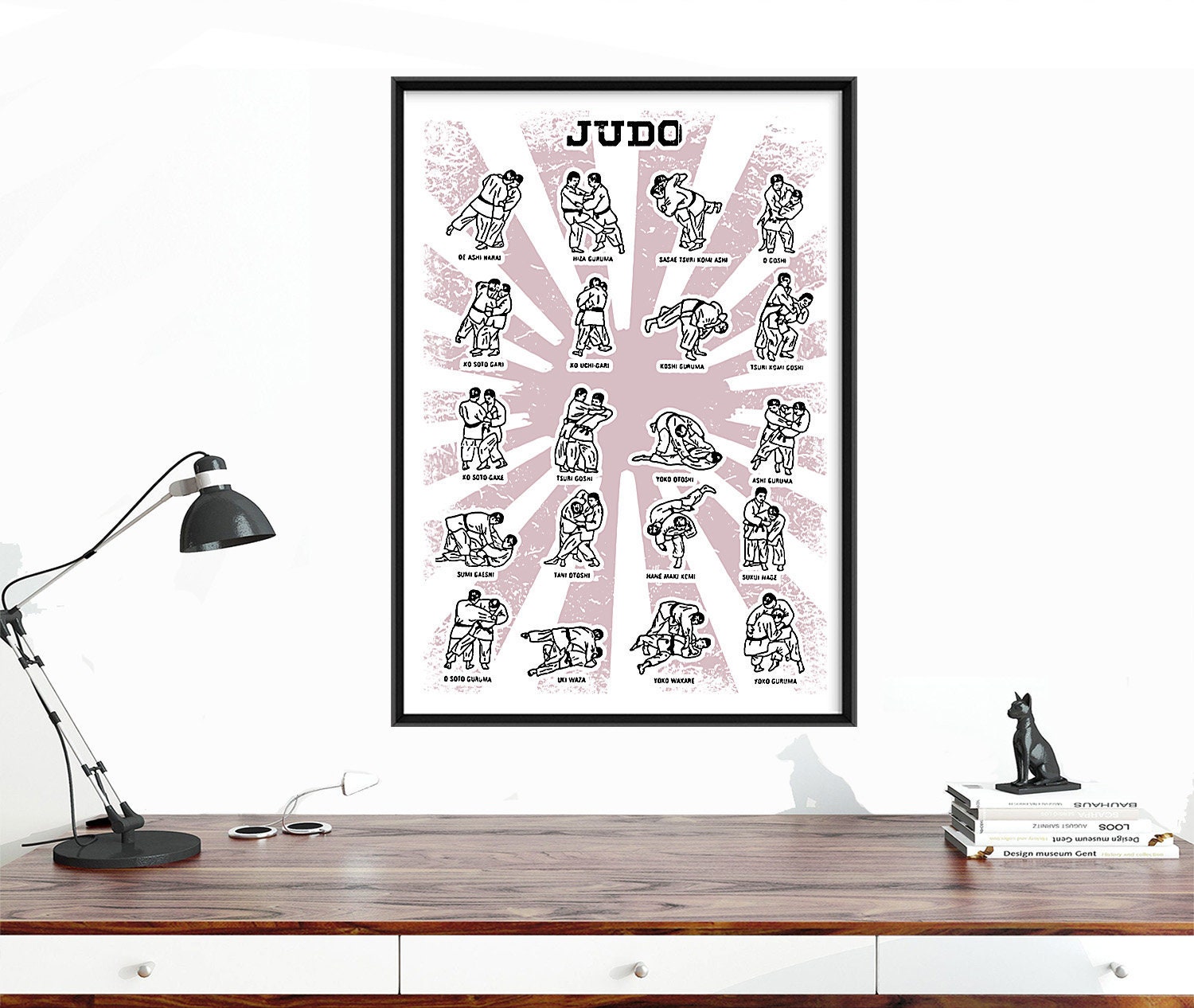The image captures a detailed interior scene featuring a desk setup and wall art. The desk, positioned towards the bottom of the photograph, has a dark wood grain top and is fitted with three white drawers. A black gooseneck lamp is stationed on the desk's left side, while the right side holds several stacked books with a small black statue—potentially a short-faced dog or cat—sitting atop them. The wall behind the desk is white and adorned with a framed poster. The poster features the word "JUDO" in bold black letters at the top and displays five rows and four columns of different Judo positions, each labeled with its name, although the specific names are not clearly visible. The background of the poster is a light purple color, resembling a radiating sun or a pink splash, enhancing the visual contrast. The overall composition of the photograph suggests a blend of function and decoration, with the workspace neatly organized and the Judo poster providing an educational and aesthetic element.